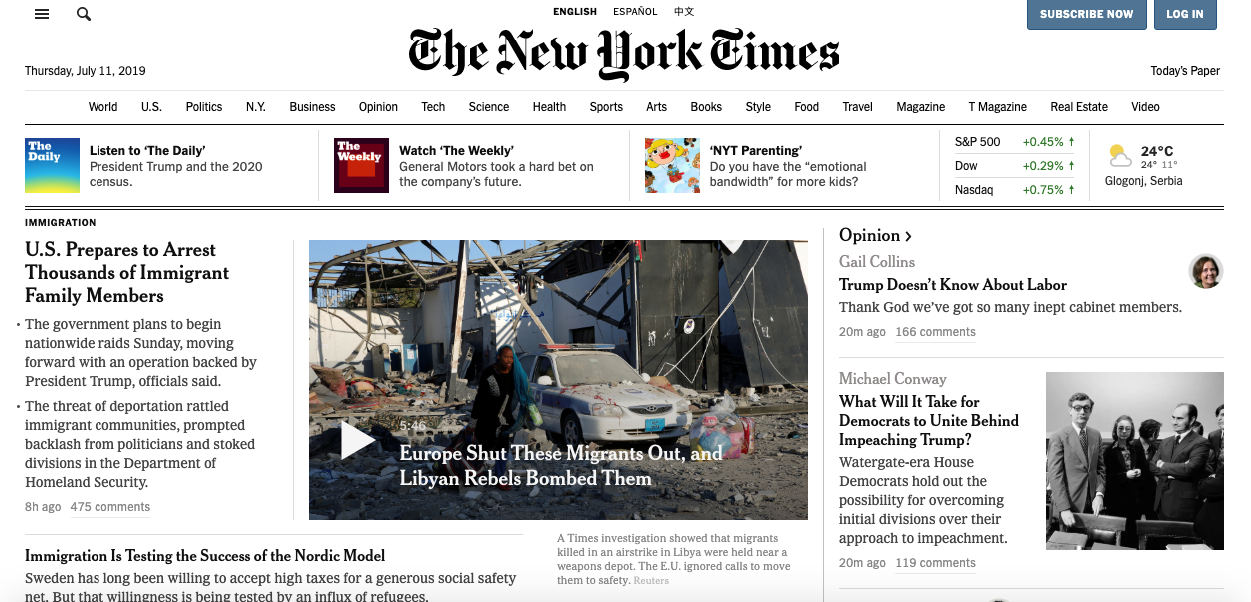Screen capture of The New York Times homepage dated Thursday, July 11, 2019. The page highlights a temperature of 24°C and features top navigation links including "Listen to The Daily," "Watch The Weekly," and "NYT Parenting." Below the navigation, various news stories are presented. A prominent video link in the center of the page reads, "Europe shut these migrants out and Libyan rebels bombed them," depicting a police car covered in dirt. Major headlines include an investigation titled "U.S. prepares to arrest thousands of immigrant family members" and an opinion piece, "Trump doesn't know about labor." Another article explores the Democratic Party’s stance with the headline, "What will it take for Democrats to unite behind impeaching Trump?" The overall tone of the articles appears to be critical of conservative politics while supporting Democratic viewpoints.